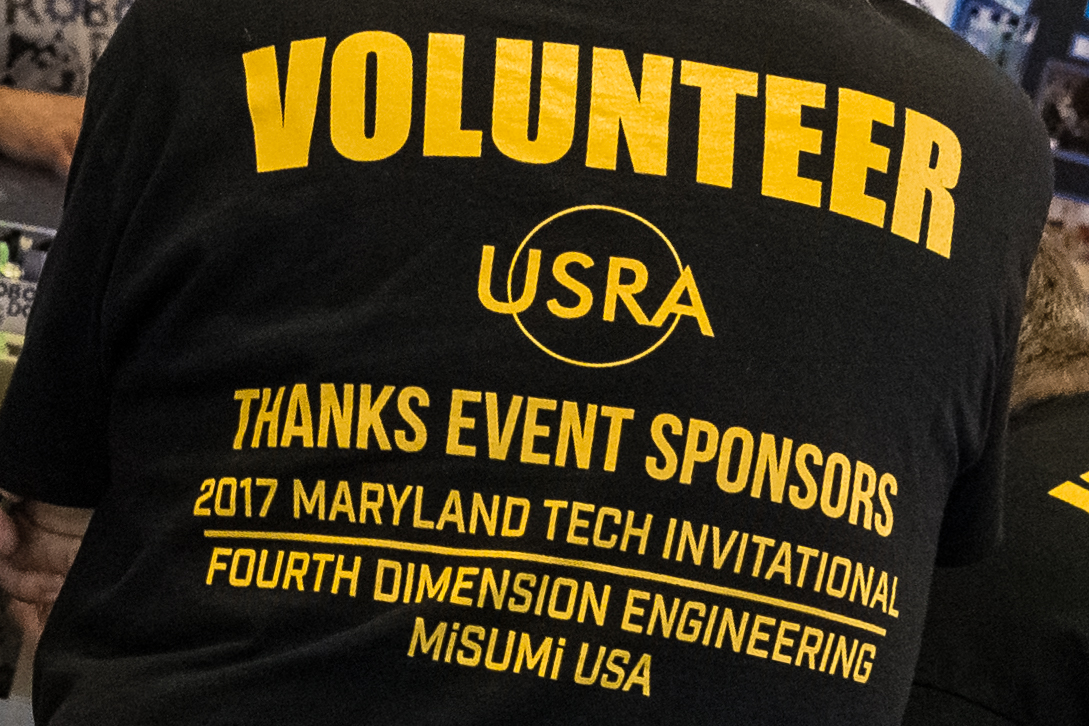The image depicts the back of an individual wearing a large black shirt. The shirt prominently features yellow text arranged in several lines. At the top, in all capital letters, it reads "VOLUNTEER," followed by "USRA" accompanied by a circular logo. Below this, the text acknowledges event sponsors with the line "THANKS EVENT SPONSORS," and specifies the event as the "2017 Maryland Tech Invitational." A yellow line separates the sponsors listed below: "4TH DIMENSION ENGINEERING" and "MISUMI USA." The person wearing the shirt is not fully visible, with only the back of the shirt in the frame.